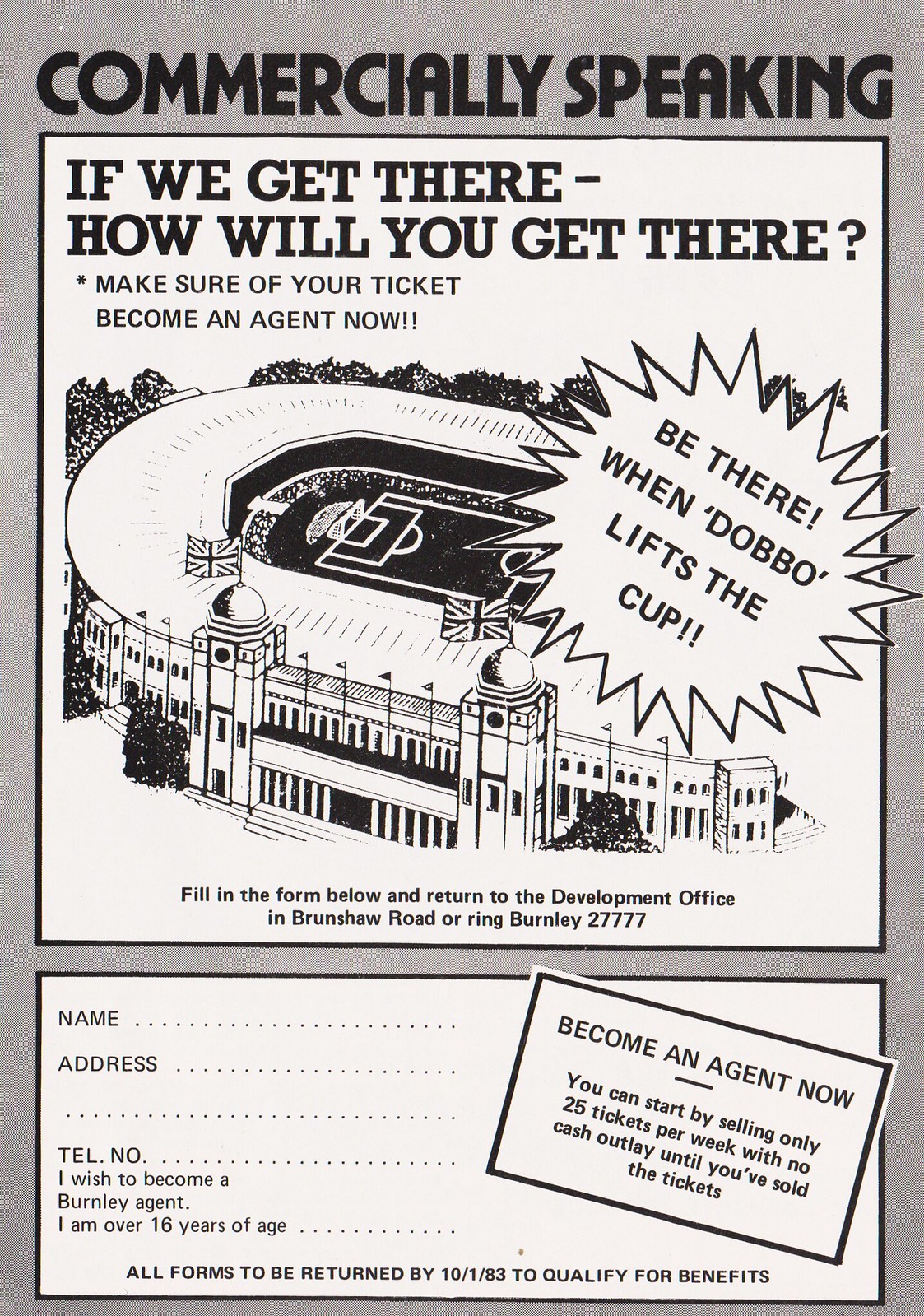The image is a vertically aligned, rectangular advertisement set against a dark gray background visible around the edges. The bold, black, all-caps title at the very top reads "COMMERCIALLY SPEAKING." Below it, a white square framed by a thin black border displays a black-and-white aerial photo of a stadium, identifiable by the soccer field and British flags on two towers at the entrance. A starburst-shaped bubble in the stadium photo proclaims, "Be there when Dabo lifts the cup." Above the image, the text prompts, "If we get there, how will you get there? Make sure of your ticket. Become an agent now." At the bottom of the advertisement, within another rectangular shape bordered in black, there is a form with dotted lines for filling in personal details such as name, address, and telephone number. The form states, "I wish to become a Burnley agent. I am over 16 years of age," and requires submissions by 10-1-83 to qualify for benefits. It instructs applicants to return the form to the development office on Brunshaw Road or call Burnley 27777.